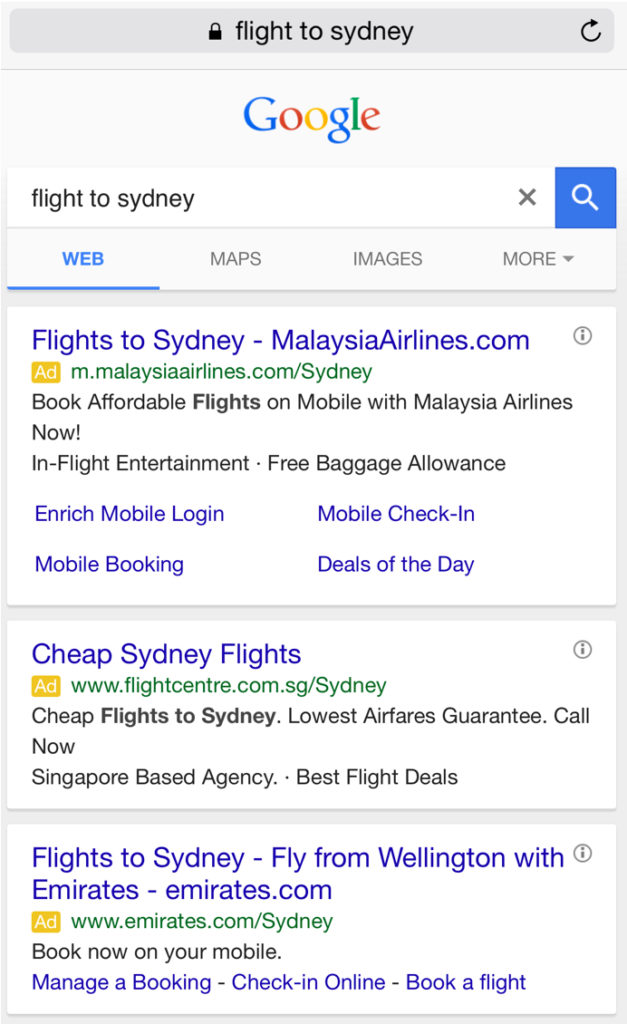This image showcases a screenshot of Google search results for the query "flight to Sydney." The image is notably tall and not very wide. 

Starting from the top, there is a dark gray rectangular toolbar that spans almost the entire width of the image, leaving thin margins on the left, right, and top edges. Within this toolbar, on the left, there is a black padlock icon indicating a secure connection. To the right of this icon, the text "flight to Sydney" is displayed. In the center of the toolbar is an empty space, and on the far right, there is a reload icon.

Below this toolbar, a fine one-pixel gray line separates it from the main content. Directly beneath this line sits the Google logo, which features letters colored in blue (G), red (o), yellow (o), blue (g), green (l), and red (e).

Next is the search bar which has the words "flight to Sydney" typed inside. At the end of this search bar, on the right, there is an 'X' button to clear the text, followed by a blue button with a white magnifying glass icon, used to initiate the search.

Underneath the search bar, there's a sub-menu for filtering search results. Currently, the "Web" filter is selected, indicated by the blue text and underline. To the right are other filter options: "Maps," "Images," and "More," which are displayed in gray.

The primary content of the image includes three different search results. These results are displayed in white rectangular blocks with blue headings, green URLs, and black descriptive text. The first result is an advertisement for Malaysia Airlines with the URL "malaysiaairlines.com/sydney." The description encourages users to "Book affordable flights on mobile with Malaysia Airlines now!" and lists features like in-flight entertainment and free baggage allowance. Below this text, there are four icons labeled: Enrich, Mobile Login, Mobile Check-in, and Mobile Booking Deals of the Day.

Below this advertisement, there are two additional search results visible, consistent in style but not detailed in this description.